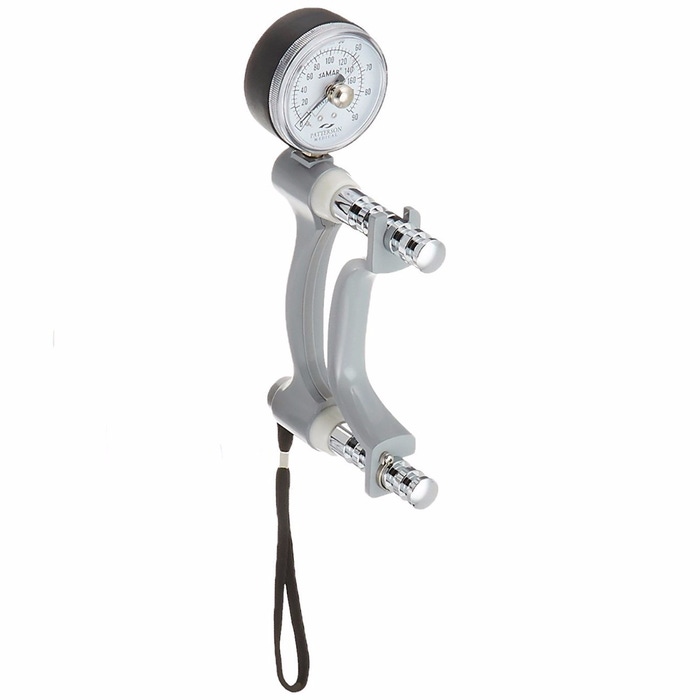This black and white photograph features a complex device that appears to be either medical or mechanical in nature. Dominating the top of the image is an analog pressure gauge with a white face, marked with numbers from zero to 160 on the inside and up to 90 on the outside. The gauge, which reads "Patterson Medical" and "Jamar" at its center, is encased in a black housing with a silver rim. Below the gauge, a robust vertical assembly features two cylindrical rods projecting outward, held together by a clamp. The device is further detailed with grey plastic and metallic elements. Additionally, a black lanyard-like string suitable for wrist attachment hangs down from the apparatus, enhancing its intricate design. The photograph is cut out against a transparent background, presenting the device in isolated white space.